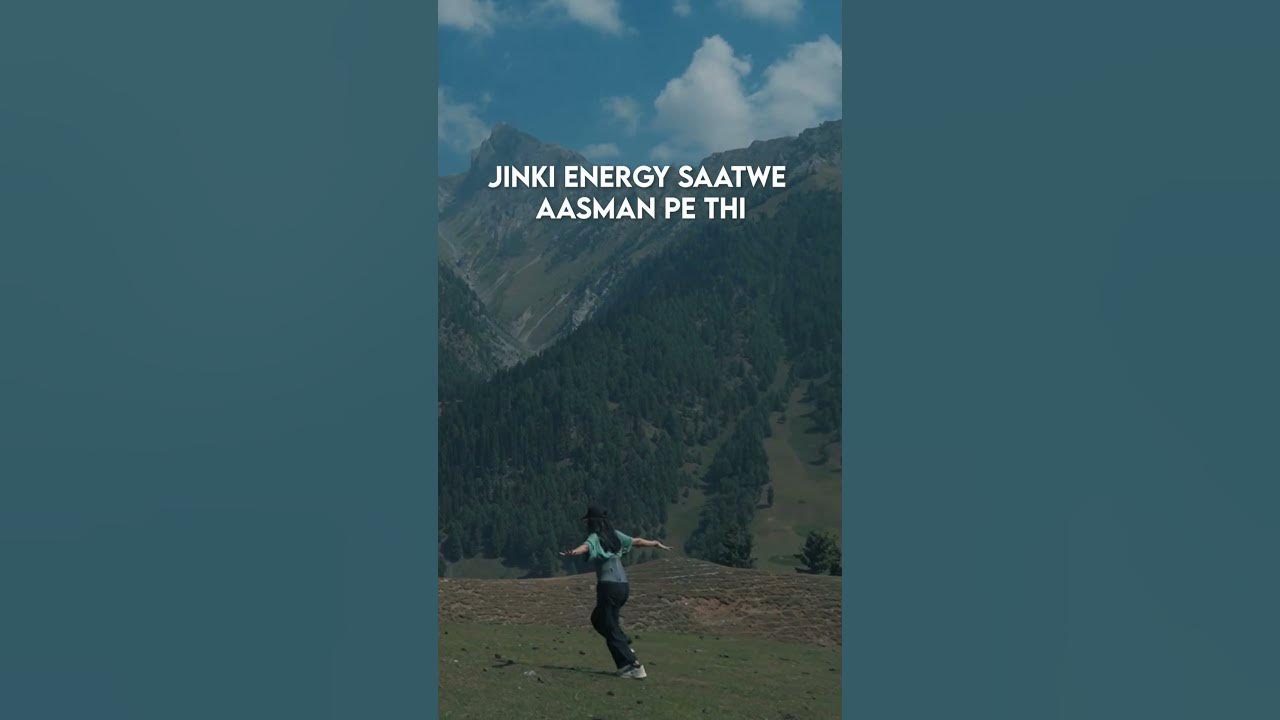The image is a color photograph presented in portrait orientation and set within a thick, dark aqua border on the left and right, forming a horizontally rectangular frame. The photograph is shot outdoors during the daytime using natural light. It captures a young woman in dark pants and a blue shirt, with long black hair, running or dancing across a grassy field. Her arms are outstretched to both sides, and she is facing away from the viewer. Behind her, tall mountains dominate the background, covered in luscious dark green pine trees, with some areas showing patches of snow. Above the mountains, the sky is a vivid blue adorned with fluffy white clouds. There is also white foreign text at the top of the photograph, spread across two centered lines. This combination of natural and digital elements, with the photographic portion featuring detailed realism, effectively communicates a scenic outdoor moment despite the poor light quality.